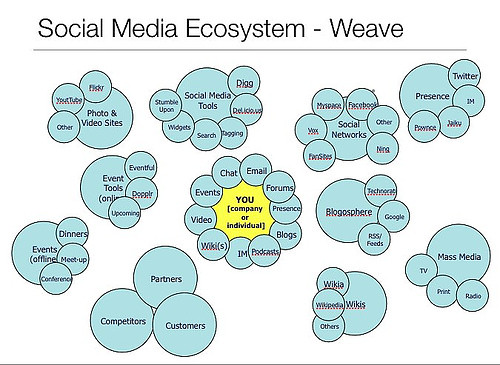The image depicts a detailed "Social Media Ecosystem - Weave" on a white background with clusters of interconnected circles primarily in light teal and a central yellow circle. At the top, in black lettering, it reads "Social Media Ecosystem - Weave," with a gray line underneath. The central yellow circle, labeled "You (Company or Individual)," is surrounded by approximately ten smaller teal circles, each representing different aspects of social interaction, including email, forums, presence, blogs, podcasts, IM, wikis, video, events, and chat. 

These smaller teal circles are linked to larger teal circles, which further categorize specific elements of the social media landscape. For example, there are clusters for "Mass Media," encompassing TV, print, and radio; "Photo and Video Sites," listing YouTube and Flickr; and other clusters such as "Social Networks," "Event Tools," and "Competitors, Partners, Customers." This intricate web visualizes the various connections and interactions between individuals or companies and the broader social media environment, demonstrating how different components such as offline events, media tools, and social networks interplay in the comprehensive social media ecosystem.